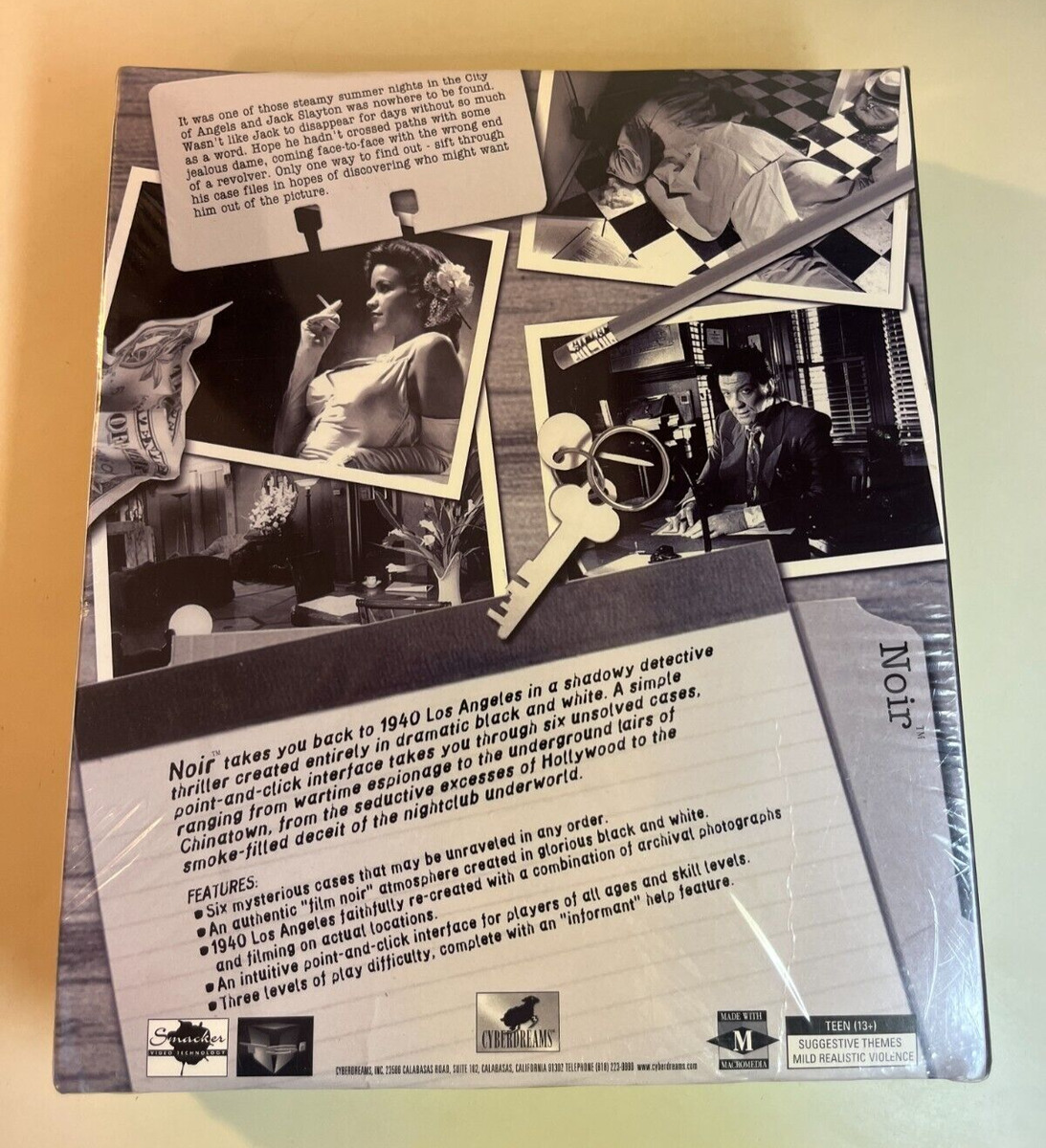This black-and-white image appears to be the back cover of a book or DVD set, capturing the gritty ambiance of a classic film noir. It is a collage of various texts and four photos arranged in a seemingly haphazard pattern, overlaid with decorative elements such as a dollar bill, a keychain, and a pencil. The text weaves a gripping tale about Jack Slayton, a detective missing during a steamy summer night in 1940s Los Angeles. It hints at the dark fates he might have met, suggesting that he could have encountered a vengeful woman and a revolver. To uncover his whereabouts, one must delve into his case files searching for clues. The background narrative promises a shadowy detective thriller set in the City of Angels, rendered in dramatic black and white.

The collage includes striking images: a woman in a sleeveless dress and mid-arm length gloves, smoking; a man in a dark suit sitting at a desk; and another man laid out face down in a suit. These visuals are tied together with the descriptive text, "Noir takes you back to 1940 Los Angeles in a shadowy detective thriller created entirely in dramatic black and white," emphasizing six unsolved cases exploring themes from wartime espionage to the underground lairs of Chinatown, Hollywood’s seductive excesses, and the deceit of the nightclub underworld. Company logos and a teen rating label indicating "suggestive themes" and "mild realistic violence" are displayed below, adding an authentic touch to this evocative portrayal of noir fiction.